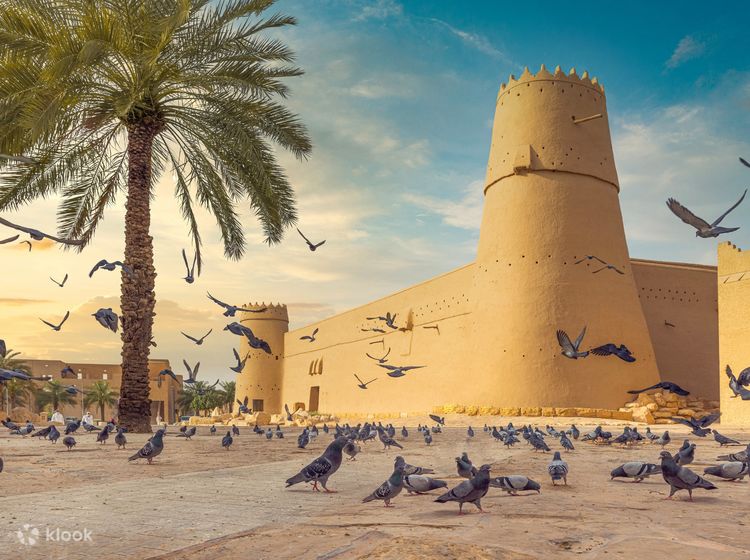The photograph captures a bustling scene in front of a large, sandy stone castle—reminiscent of Middle Eastern architecture—set against a bright, partly cloudy blue sky. The castle, with its slightly sloped round towers and solid walls, stretches across the right two-thirds of the image, exhibiting a vibrant limestone-yellow color that glows warmly, especially around what appears to be late afternoon or sundown. This photorealistic scene is teeming with activity, with numerous gray pigeons, adorned with darker gray and black markings, flocking both on the sandy gravel pathway below and in mid-flight. A prominent green palm tree with a rough brown trunk stands on the left, occupying roughly a third of the image, enhancing the desert ambiance. In the distance, partially obscured by this tree, is another two-story building, linked visually to the castle, and dressed in white, hinting at further historical or architectural significance. The scene includes additional details such as small holes in the castle walls, possibly for visibility or ventilation, and a straight rod protruding from one of the towers, suggesting possible modern interventions. The photograph also includes a white, transparent watermark in the lower left corner reading "KLOOK".